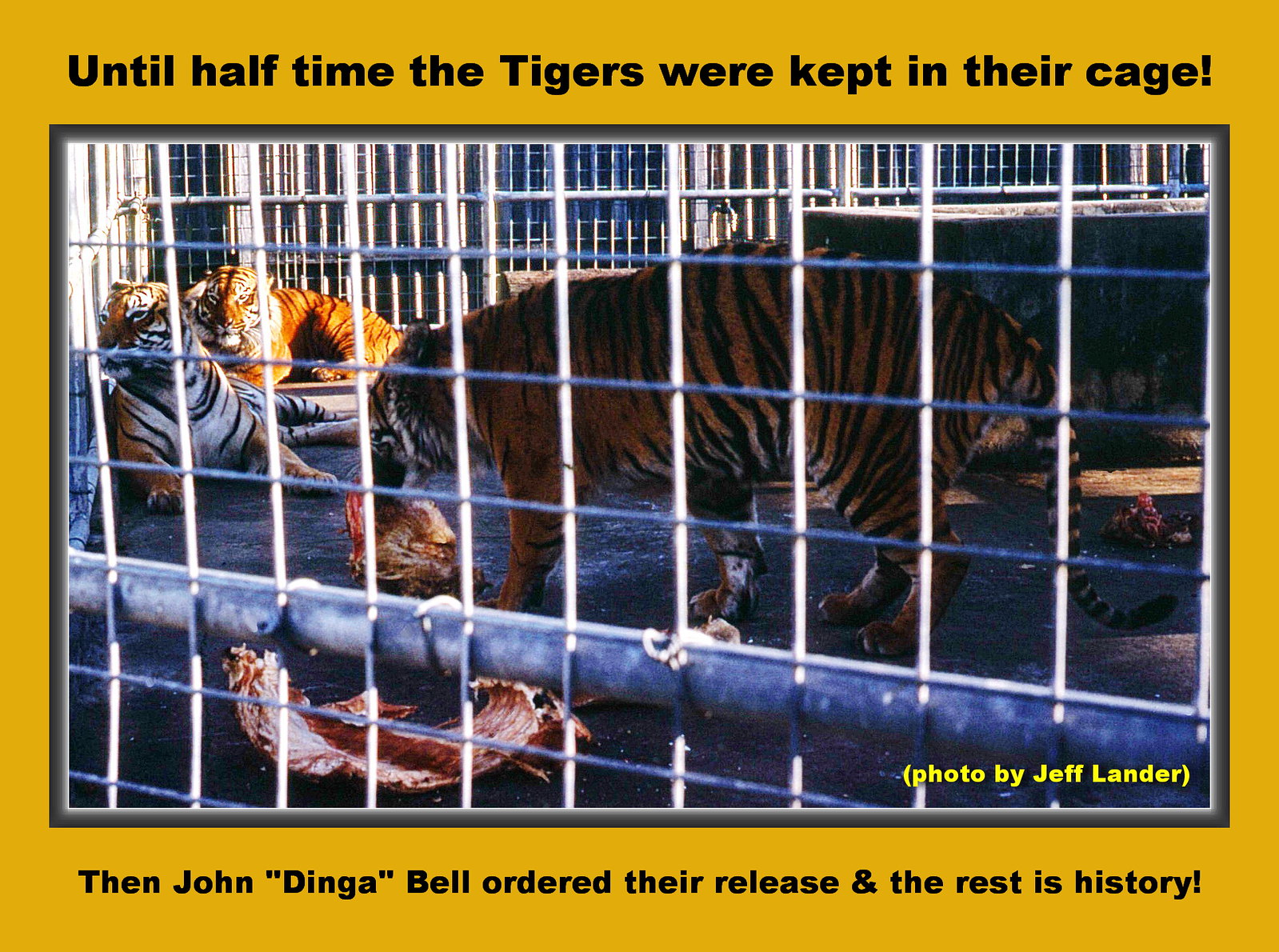This wide rectangular image, encased in a deep yellow digital frame with thicker borders at the top and bottom, vividly captures a dramatic moment involving tigers. At the top of the frame, bold black letters declare, "Until halftime the tigers were kept in their cage!" The bottom text states, "Then John 'Dinga' Bell ordered their release and the rest is history!" Additionally, in the bottom-right corner of the frame, yellow text reads, "Photo by Jeff Lander."

The central photograph, taken from behind a grid of thin silver metal bars, reveals a zoo-like exhibit with a concrete floor littered with meat scraps. Inside the cage, three tigers are visible: one stands facing left, seemingly alert, while two others lay in a corner near the top left of the image, bathed in sunlight and looking to the left. One of the tigers is seen eating a piece of meat, adding to the scene's dynamic and raw atmosphere. The detailed setup, vivid descriptions, and striking imagery create a compelling and thorough visual narrative.